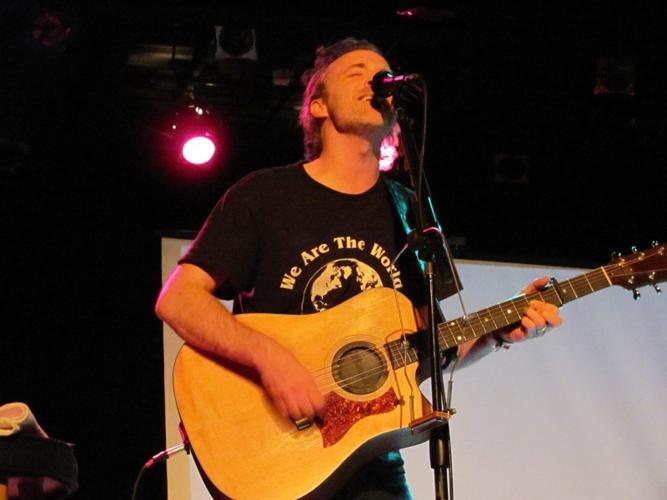In this photograph, a guitar player is immersed in his performance onstage. The background is predominantly black, aside from the subtle illumination by purplish lights coming from the rafters. These lights create an ethereal glow around him, even tinting his hair with a hint of pink. A faint bluish-green light near him gives his sleeves a slight greenish hue. The stage is minimal, with a large gray screen or perhaps a white sheet behind him adding a contrasting backdrop to his figure.

He's in the midst of a song, standing with a black microphone stand right at his mouth. His head is tilted back, eyes closed, and a slight, serene smile graces his face, showing his deep connection to the music. He is dressed in dark-colored pants and a black t-shirt that prominently features the phrase "We Are The World" above an image of a globe. 

With a confident stance, he strums a wooden-faced guitar with a darker wood neck, both hands engaged in creating music. A cord extends from the guitar, hinting at the electrifying sound he's producing. The combination of his relaxed yet energetic posture and the powerful lights makes for a captivating scene that underscores his passion and the ambiance of the concert environment.